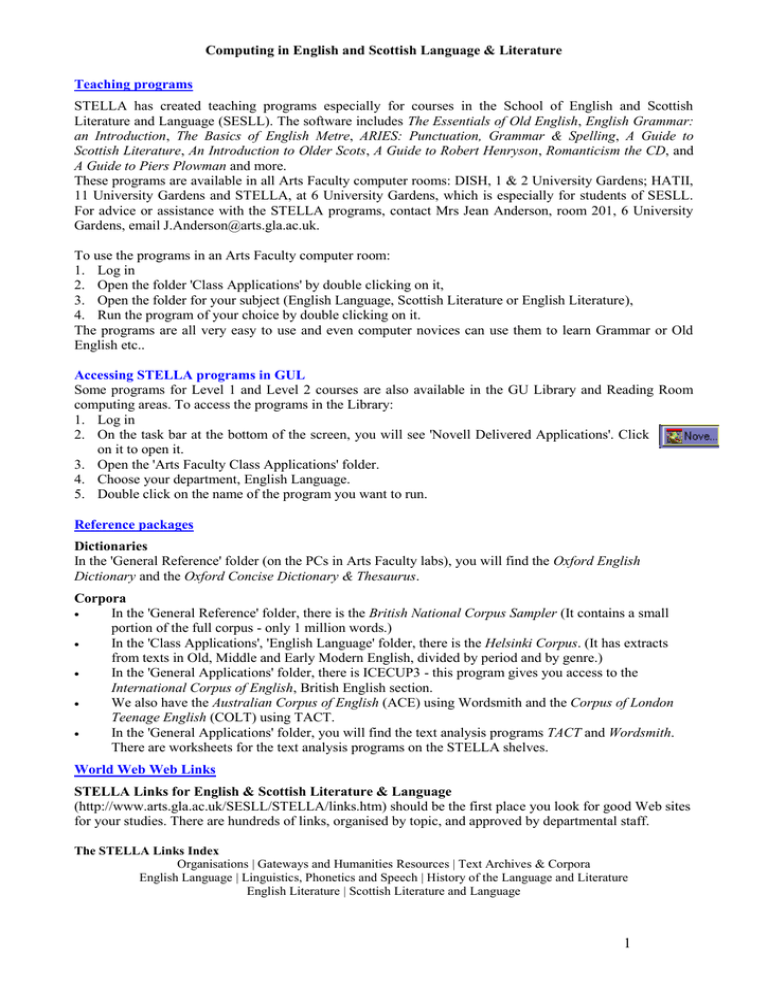The image features a detailed informational poster divided into several sections with different colored texts and backgrounds to enhance readability.

**Top Section:**
- The top part of the poster has a white background with the title "Computing: English and Scottish Language and Literature."
- Below the title, a blue underline highlights the subheading "Teaching Programs."

**Main Body:**
- The primary text, in black font, reads: "Estella has created teaching programs specifically for courses in the School of English and Scottish Literature and Language (SESLL). These programs include essentials on Old English, English Grammar, Scottish Literature, and Introduction to Older Scots. Additionally, it provides guides to topics such as Robin Henry's Romanticism and a CD guide to Pierce, Plummer, and more. The programs are accessible in all Arts Faculty Computer Rooms at Dish, 1 and 2 University Gardens, HALF, 11 University Gardens, and particularly at 6 University Gardens for SESLL students. For advice or assistance with Estella programs, contact Mrs. Jean Anderson in Room 201 at 6 University Gardens. Email: j.anderson@arts.ga.ac.uk."

**Step-by-Step Instructions:**
- Another section in black text provides detailed steps for using the programs in the Arts Faculty Computer Room:
  1. Log in.
  2. Open the "Class Application" folder by double-clicking on it.
  3. Open the folder for your subject (English Language, Scottish Literature, or English Literature).
  4. Run a program of your choice by double-clicking on it. The programs are user-friendly, even for computer novices.

**Highlighted Sections:**
- A segment with a blue background and blue font instructs users on how to "Access Estella Programs in Gaul."
- The bottom portion features two sections with blue backgrounds titled "Reference Packages" and "Worldwide Web Links," presumably listing additional resources and relevant websites.

This detailed caption provides a comprehensive understanding of the poster’s content and instructions, making it easier for users to navigate and utilize the Estella teaching programs.